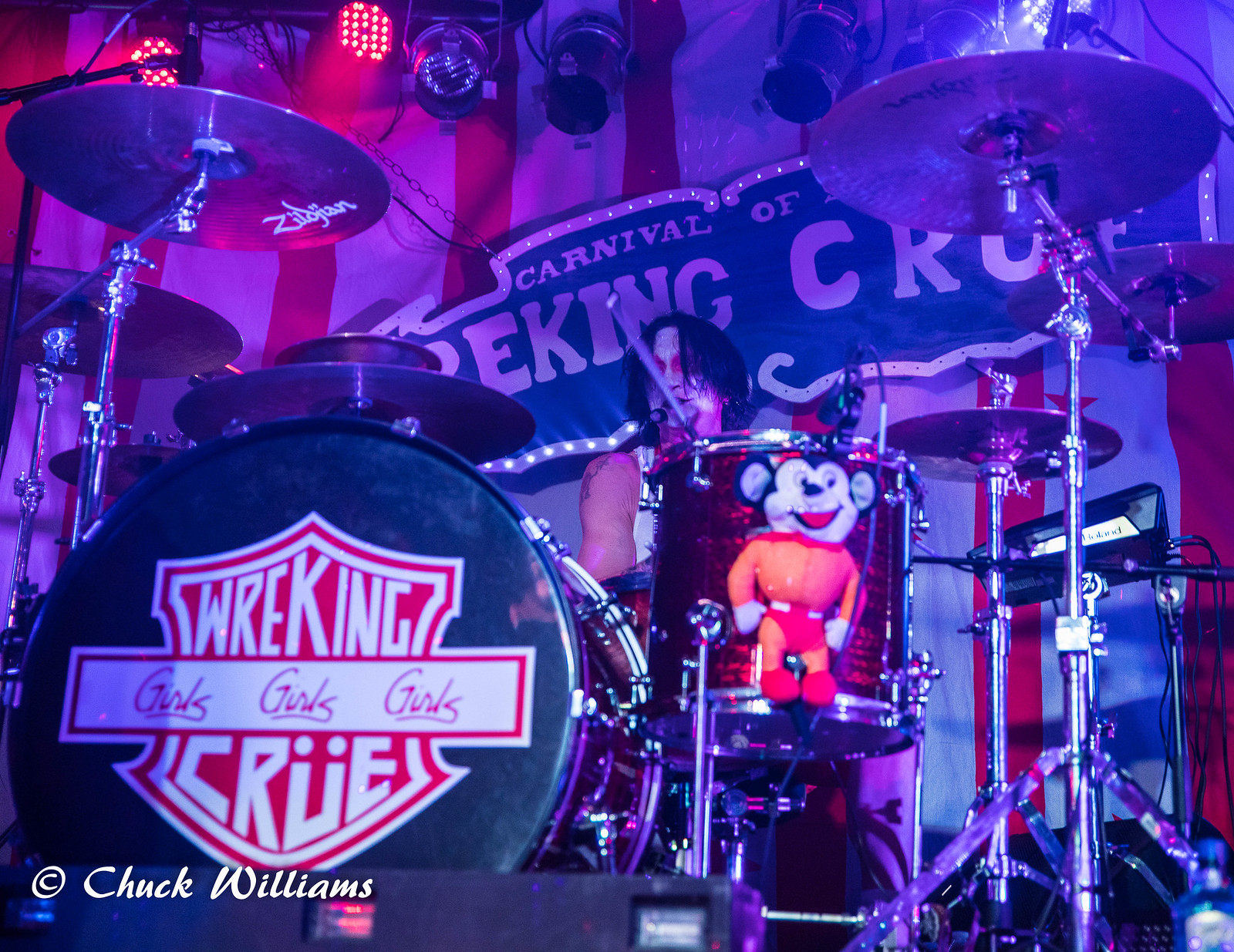The image portrays a dynamic stage performance featuring a drummer, potentially Tommy Lee from Mötley Crüe, engrossed in his drum set. He is adorned with theatrical white face paint, black lipstick, and shoulder-length black hair partially obscuring his eyes, wearing rose-colored sunglasses. The drummer is captured mid-action, with one drumstick raised near his face. He is surrounded by a heavy assembly of various cymbals and drums, supported by silver stands, with visible wires and spotlights accentuating the dramatic atmosphere—two spotlights are red, and one is blue.

Central to the stage is a distinctive black bass drum featuring a prominent red and white logo that reads "Wrecking Crew," embellished with dual dots over the 'U,' and the phrase "Girls, Girls, Girls" emblazoned below it. Attached to the red snare drum directly in front of him is a stuffed doll resembling Mickey Mouse, dressed in an orange outfit. The backdrop is vivid with red and white stripes resembling a circus tent, contributing to the carnival-like ambiance of the set. Obscured text hints at "Carnival of," augmenting the thematic setting. In the bottom left corner, a copyright symbol and the name "Chuck Williams" are visible, attributing the photograph.